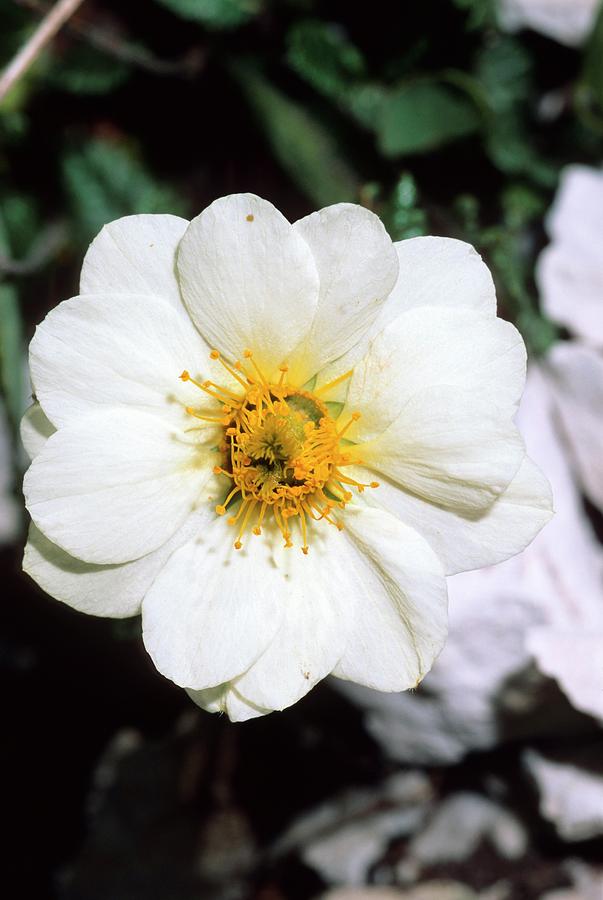The image presents a stunning close-up of a blooming Mountain Evans flower, belonging to the rose family. The central focus is a white flower with smooth, overlapping petals that form a cluster-like arrangement around its yellow center. Numerous yellow stamens project from the center, casting delicate shadows on the pristine white petals, further emphasized by the sunlight's glow. The background features a blurred array of leaves and other flowers, predominantly in shades of green and white, creating a soft and natural ambiance. The flower, positioned prominently in the middle of the frame, exudes a sense of tranquility and highlights the intricate beauty of nature's design. The entire composition, captured outdoors in natural lighting, epitomizes the serene elegance of botanical photography.